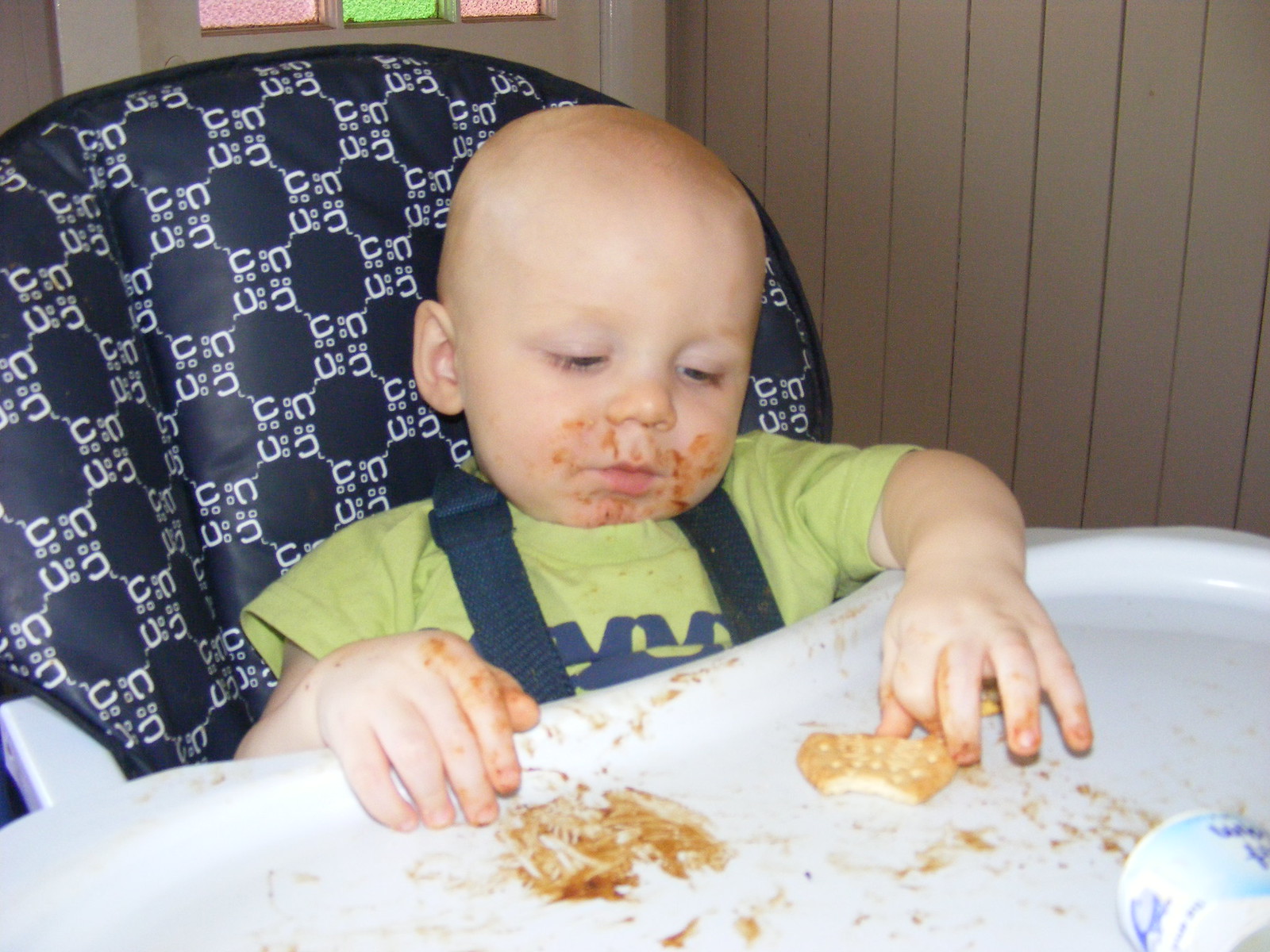The photograph captures a close-up scene of a young toddler, around one to two years old, sitting in a high chair. The child, with short, light-colored hair, is messily eating, evident by the brown sauce smeared all over their face and hands. The baby is wearing a green shirt with blue writing on it. The white plastic tray of the high chair is cluttered with food remnants, including a partially eaten light brown cracker. The chair's cushion features a dark blue checkered pattern with white sea and bubble shapes forming letter C squares. Behind the toddler, the walls are painted a light tan color, and there is a door with stained glass panels in shades of pink and green.